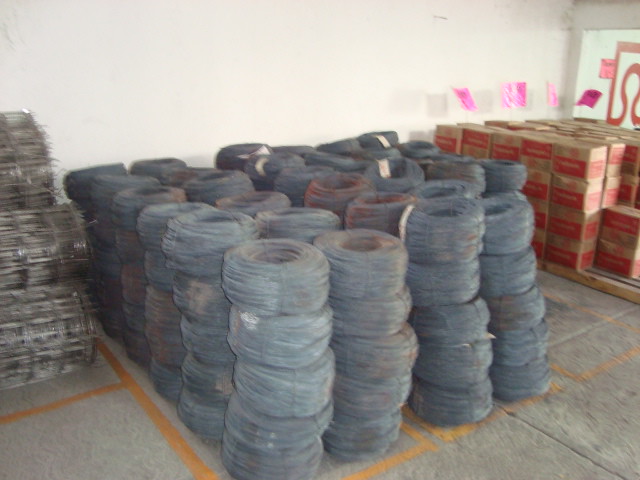In this image, we see what appears to be a spacious industrial garage or warehouse with a concrete floor marked by solid yellow lines. The central focus of the picture is stacks of coiled materials, possibly tires, hoses, or wires, organized in neat rows about four coils wide and extending six stacks deep towards the back of the space. To the right side of the image, there are numerous large brown cardboard boxes with red markings on them, accompanied by pink papers positioned above. On the left side, a rolled-up metal gate adds to the industrial ambiance of the setting. The meticulously arranged elements and the vast, organized open area suggest this space is used for storage or maintenance purposes, possibly for a business dealing in automotive parts or similar equipment.